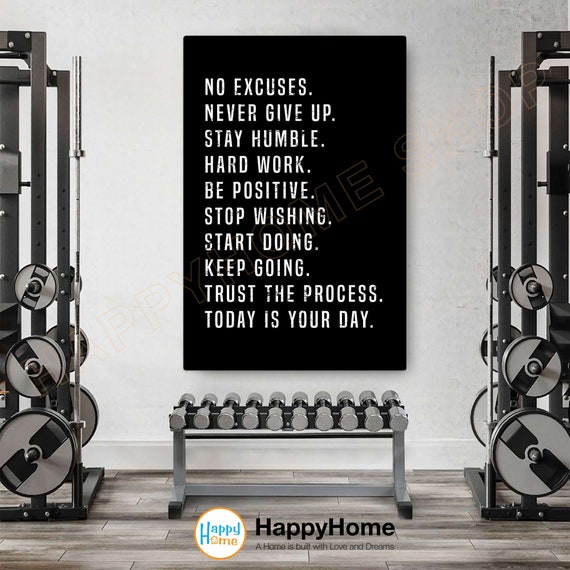In this black-and-white gym photograph, a striking white wall serves as the backdrop for a large black sign featuring an array of motivational phrases in white text: "No excuses, never give up, stay humble, hard work, be positive, stop wishing, start doing, keep going, trust the process, today is your day." Below the sign is a well-organized rack of shiny silver dumbbells, neatly arranged from the lightest on the left to the heaviest on the right. Adjacent to the rack on both the left and right sides are two tall fitness machines, likely lat pull-down machines, with visible weights at the back, which are also silver in color. The gym floor is composed of a beige-gray wooden texture, adding warmth to the monochrome decor. At the very bottom of the sign, the text "Happy Home" appears, though the text beneath it is too small to be legible. The entire scene exudes a determined and encouraging atmosphere, perfect for motivating gym-goers.